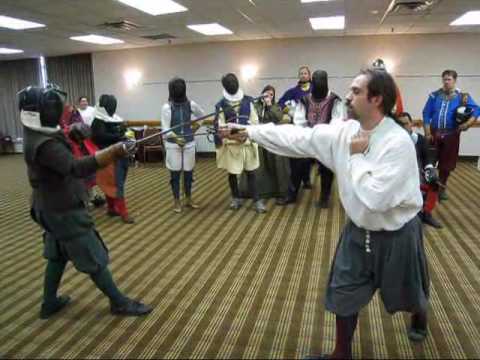In this small horizontal rectangular image, we see a scene resembling a medieval fighting class taking place in a well-lit, carpeted room, which looks akin to a conference room. In the foreground, two individuals are engaged in a mock sword fight with non-lethal swords, likely for training or demonstration purposes. The man on the right wears a white long shirt paired with black trousers, while the person on the left, whose gender is not clearly identifiable, dons similar pants and a black shirt with a black helmet, along with black socks and shoes. Both are outfitted in attire reminiscent of medieval times, including a white ruffle around the neck for the individual on the left. The setting features striped carpeting in hues of yellow and dark brownish-green, and the ceiling is lined with fluorescent lights. Behind these two, several other participants, dressed similarly with some wearing traditional fencing helmets, observe the sparring session. This group, standing against the white walls of the room, contributes to the ambiance of a disciplined yet historical martial arts practice.